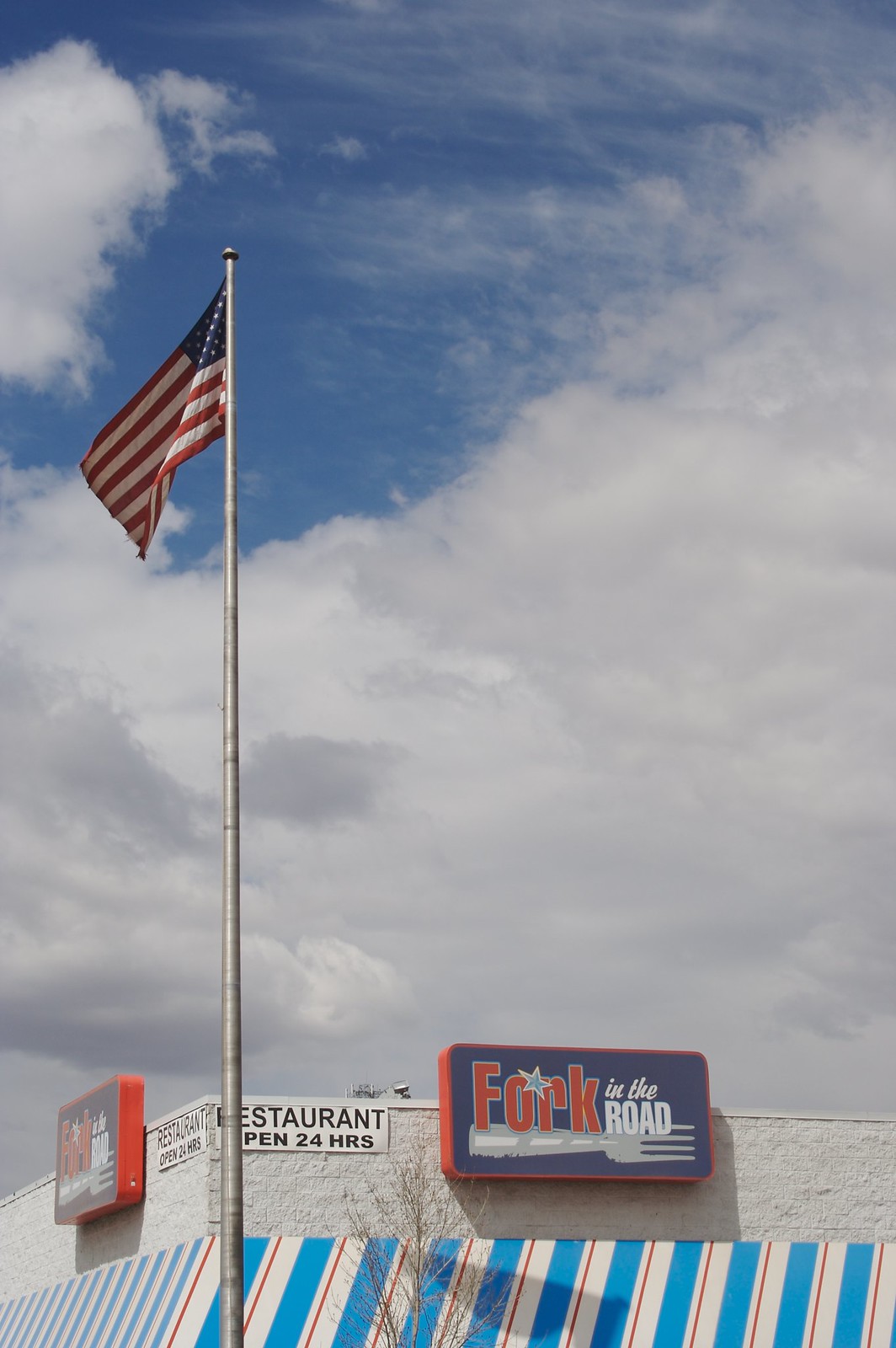The image captures a vibrant scene with a striking sky taking up the top half, filled with heavy white and light grey clouds, through which patches of blue peek through. Dominating the left side of the image is a tall, silver pole topped with an American flag, which is blowing to the left, showcasing its red and white horizontal stripes and a blue square studded with white stars. Below the flag, there stands a white-painted brick building adorned with an awning that features diagonal blue, red, and white stripes. Prominently displayed on the building's corner is a white sign that reads "Restaurant Open 24 Hours." Above this, a red and blue sign with the text "Fork in the Road" stands out, with the words "Fork" and "in the Road" written in white, and a star featured prominently on the sign. A small, leafless tree is situated at the bottom center of the image, near the building, adding to the detailed composition of the photograph.